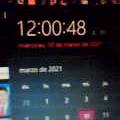The image features a detailed snapshot of a digital calendar and clock display. At the top of the image, the current time is prominently shown as "12:00:48," complete with running seconds. Below this time display, the calendar is set to March 2021. The days of the week are listed horizontally, and beneath them, the dates are shown. The first visible row of dates includes "30, 1, 2, 3, 4," while underneath them, the next row displays "7, 8, 9, 10, 11." The remaining calendar days and details may extend beyond the frame of the image.